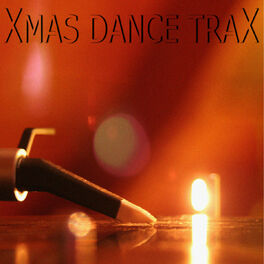The image depicts what appears to be an album cover for a CD titled "XMAS Dance TRAX," specifically showcasing Christmas holiday dance music. The album title is featured at the top, spelled out in a transparent font outlined with black shadows, making "XMAS Dance TRAX" legible. The cover showcases a highly zoomed-in, macro shot dominated by warm hues, predominantly in shades of red, orange, and yellow, giving the cover a festive yet unconventional vibe. Central to the image is a metallic handle with a softer cloth-like extension, suggestive of an ambiguous object. The handle and the cloth are positioned against a shiny reflective surface, possibly resembling a disc player's needle setup. The bottom right of the image features a prominent bright yellow light, reflected off the shiny surface, hinting at a background light source that contributes to the overall warm color scheme. The festive and abstract nature of the design ties into the dance-oriented holiday theme, even though it deviates from traditional Christmas imagery.